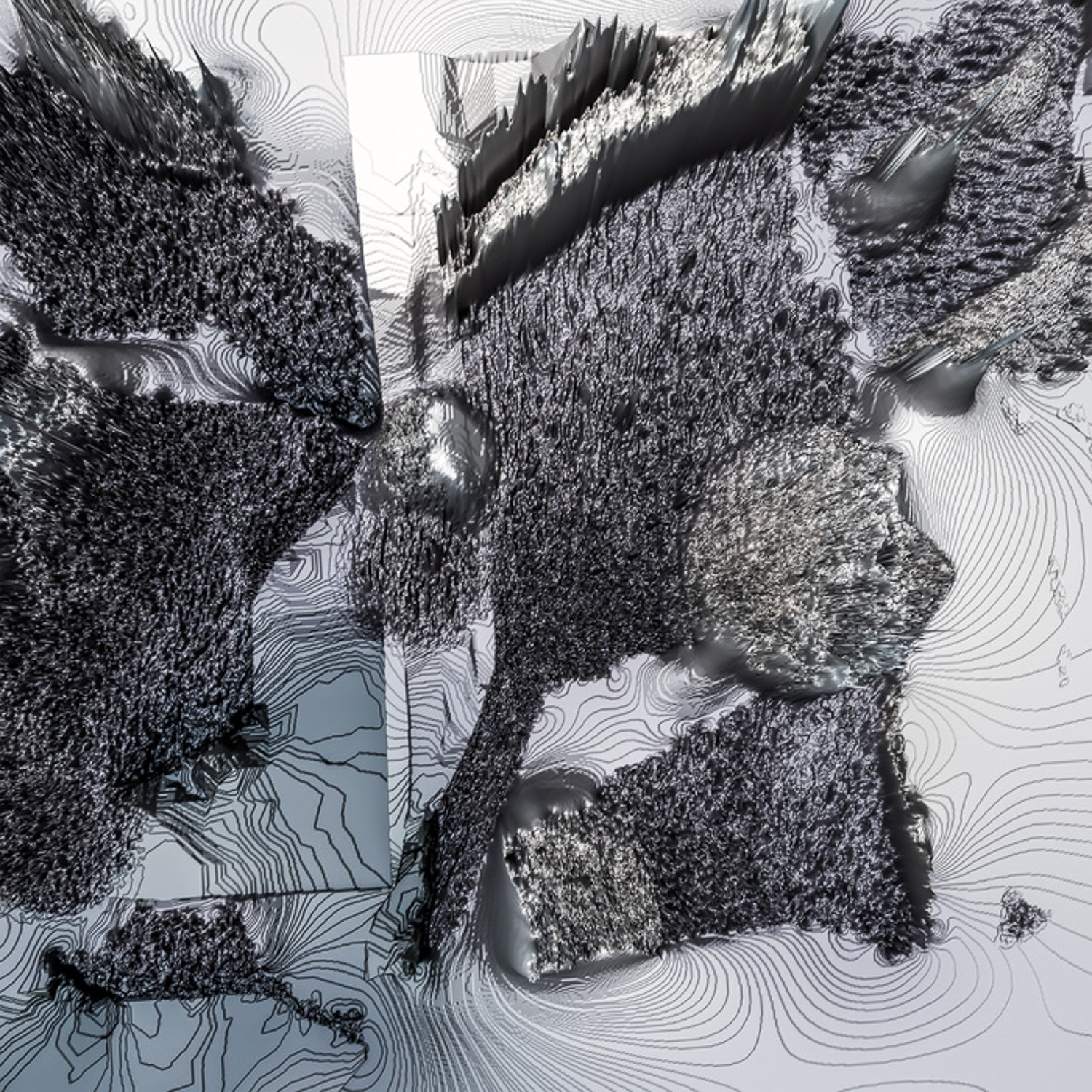This intriguing black and white image presents an abstract composition that evokes various interpretations. It resembles an aerial, bird's-eye view of a strange, map-like landscape. In the center, an area that seems to embody dark, moss-like vegetation spreads out, surrounded by intricate, squiggly lines akin to water or topographical map contour lines. These squiggles, appearing like swirling patterns on paper, lend a cartographic quality to the piece. Shadows and gradients enrich the scene, with a notably darker gray background in the bottom left corner. Additionally, some observers interpret a torn-up stuffed animal laying across this landscape, with recognizable features such as a head, striped back or tail, and an ambiguous piece of plastic in the top left. The overall effect is a highly detailed, grayscale image that blurs the lines between a detailed drawing, an art installation, and an abstract representation of a landscape.